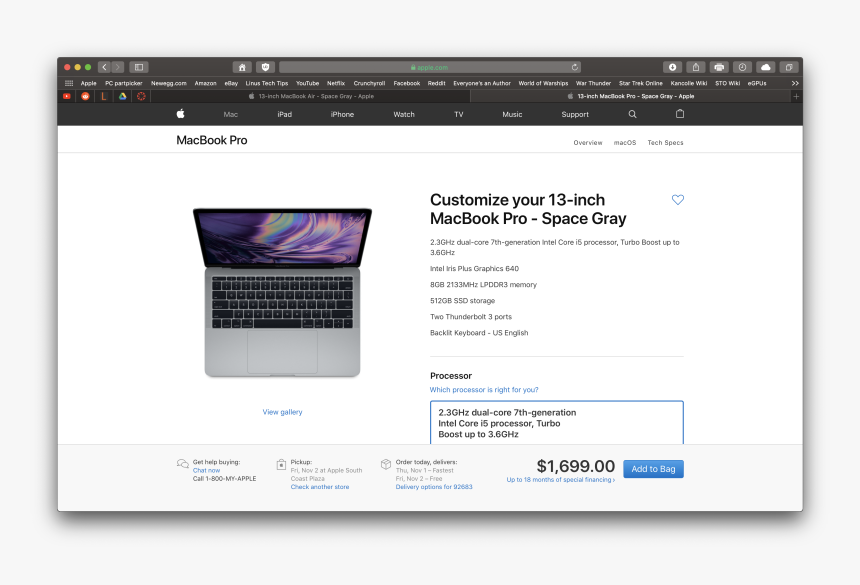A person is viewing the Apple website on a MacBook. The screen clearly shows the typical macOS window elements: a green, yellow, and red dot in the top left corner, indicating the minimize, maximize, and close functions. To the right of these dots, there are navigation arrows—backwards and forwards—encased in light gray, rounded squares, with the forward arrow disabled.

On the webpage, the upper left area features a white Apple logo set against a dark gray strip. Adjacent to the logo, the navigation options are listed: 'Mac' in light gray text, followed by 'iPad,' 'iPhone,' 'Watch,' 'TV,' 'Music,' and 'Support' in white text. There are also search and shopping cart icons in this strip.

Dominating the page is a bold, black headline that reads “MacBook Pro” on a white background. To the right of this headline are three sections of text, with the middle section clearly stating "macOS." Below, a featured image of a MacBook Pro showcases a vibrant wallpaper with abstract colors in green, blue, purple, and pink. The laptop itself is light gray, with black keys and lettering that appears to be either light gray or white.

Further to the right, there’s text that reads, "Customize your 13-inch MacBook Pro - Space Gray," next to a blue-outlined heart icon. Below this, specifications of the laptop are detailed, including a bold heading stating "Processor." The text indicates a 2.3 GHz dual-core seventh-generation Intel Core i5 processor, with a turbo boost capability of up to 3.60 GHz.